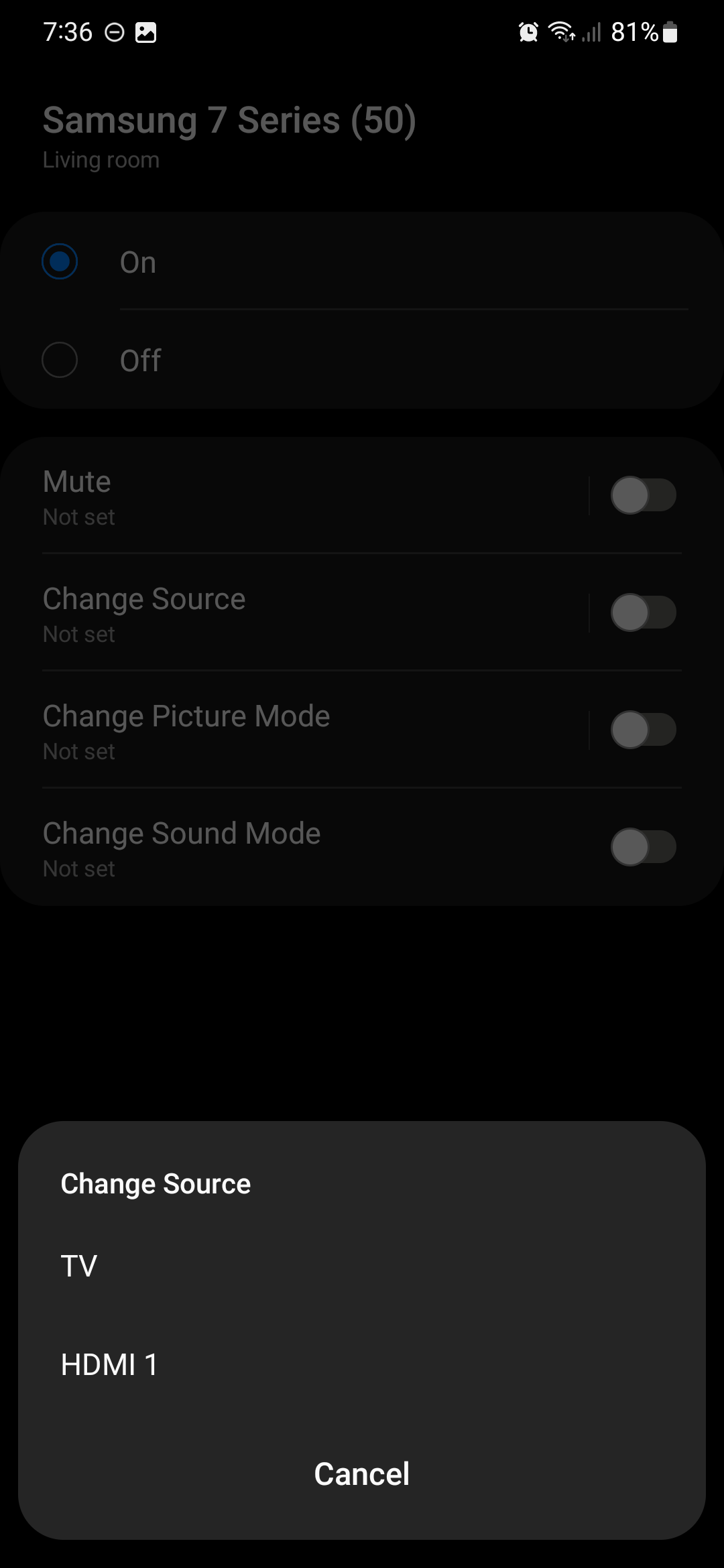This screenshot, captured from a mobile device, showcases a user interface with a black background. Along the top, a series of white icons display common mobile indicators, including time, Do Not Disturb status, notifications, alarm clock, Wi-Fi connection, network signal strength, and battery status.

At the bottom of the image, there is a lighter-toned pop-up box that stands out against the darker background. This box provides details for setting up a connection, possibly between a phone and a TV or another device. Displayed prominently is the device name, "Samsung 7 Series Living Room," with a selected radio button indicating the connection is active.

Below the device name, there are four additional options: Mute, Change Source, Change Picture Mode, and Change Sound Mode. Each of these options is accompanied by a slider button, all of which are currently switched off. Towards the bottom of the pop-up box, the "Change Source" option reveals two available selections: "TV" and "HDMI 1." The interface also includes a "Cancel" button for exiting this configuration screen.